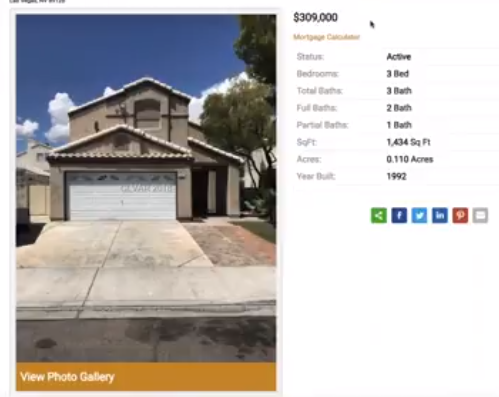This image is a partial screenshot of a house listing. The upper left-hand corner is partially cut off, making some of the text illegible. The left side of the image displays a photograph of the house taken from the road, leading up the driveway. The right side contains detailed information about the house listing.

On the right side:

- The asking price is prominently displayed as $309,000 in bold black text.
- Below the price, there is an orange link labeled "Mortgage Calculator."
- A black cursor is visible, suggesting the screenshot was taken while browsing the listing.
- Below this, in a gray column, are various categories for the house’s description, with corresponding details in black text:
  - Status: Active
  - Bedrooms: 3 Beds
  - Total Baths: 3 Baths
  - Full Baths: 2 Baths
  - Partial Baths: 1 Bath
  - Square Footage: 1,434 Sq. Ft.
  - Acres: 0.110 Acres
  - Year Built: 1992

Beneath these details, aligned to the right, are several social media icons for sharing the listing:
- Generic share icon (green)
- Facebook (white "F" on a blue square)
- Twitter (white bird on a light blue background)
- LinkedIn (white "IN" on a dark blue background)
- Pinterest (white "P" on a red background)
- An email icon depicted as a gray rectangle with a horizontal line through the middle.

At the bottom of the picture is a link with white text on an orange background banner that reads "View Photo Gallery."

The main image shows a two-story house with the following details:
- A two-car garage with a white, four-part metal door featuring a handle in the middle.
- Decorative scalloped arches across the top of the garage door, forming a pattern of four arches.
- The garage roof is tiled, which is evident from the edges and a peak visible over the roof.
- The rest of the house extends behind the garage, with three distinct roof lines – one on the left and two on the right, which could be a perspective issue or an actual differentiation in roof design.
- The main entrance appears to be on the right side of the garage, indicated by a paved area that resembles an entryway, though no door is visible.
- Short trees are planted on the right side of the house, extending out of the frame. Possible structures, such as a neighbor's house or accessory buildings, are visible behind these trees, though they are not clearly defined.
- The left side of the image shows another house, possibly in a similar style, set further back from the road. It's unclear if the visible garage or building belongs to this property or the neighboring one.

The sky above is mostly clear with some clouds on the low horizon, set against a bright blue backdrop.